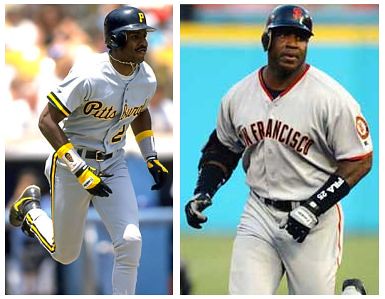This image is a side-by-side composition of two photographs separated by a white line, featuring the same baseball player, likely Barry Bonds, in different uniforms representing two teams. In the left photograph, the player is captured mid-run towards the right. He dons a Pittsburgh Pirates gray button-up baseball jersey emblazoned with "PITTSBURGH" in black font with a yellow border across the chest and the number 2 on the front. The jersey sleeves end in yellow stripes. He pairs the jersey with matching gray pants that feature a yellow stripe bordered by black lines along the sides, and completes the look with a black belt with a silver buckle. His black cleats have yellow trim. A blue helmet with a yellow "P" adorns his head, and he appears to be wearing a necklace.

The right photograph shows the same player, now in a different uniform, representative of the San Francisco Giants. "San Francisco" is inscribed on his chest in red and black writing. He wears a black batting helmet featuring the San Francisco logo, black batting gloves, and wristbands. In this image, he appears to be walking and his left leg is in mid-motion, highlighting the dynamic moments in each photograph. The background in both photos is blurred, emphasizing the player and his distinct uniforms.